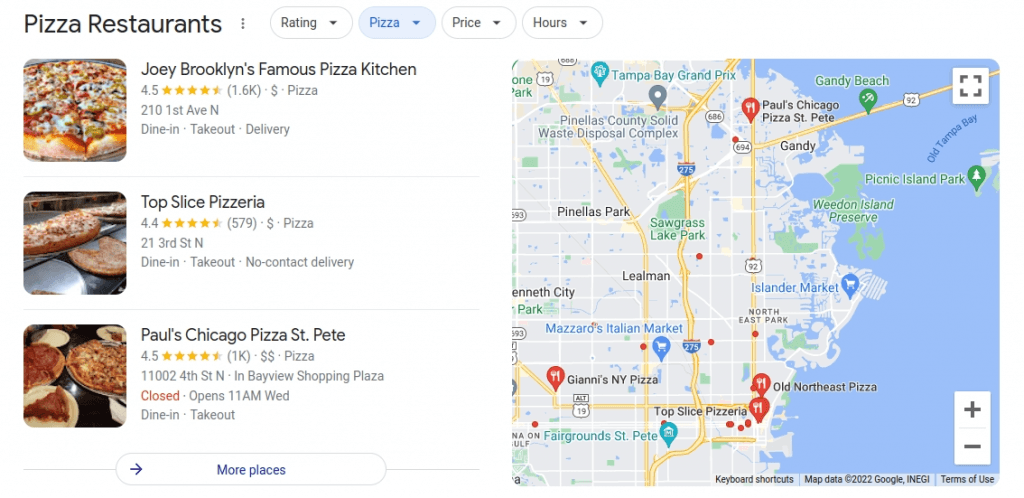A detailed screenshot on Google Maps depicts a search for pizza restaurants, likely in Florida, as evidenced by local landmarks such as the Tampa Bay Grand Prix and Fairgrounds St. Pete. Three notable pizza restaurants are listed with their ratings, reviews, and operational details:

1. **Joey Brooklyn's Famous Pizza Kitchen**
   - **Rating:** 4.5 stars
   - **Reviews:** 1.6k
   - **Price:** $
   - **Services:** Dine-in, take-out, delivery
   - **Location:** 210 First Avenue North

2. **Top Slice Pizzeria**
   - **Rating:** 4.4 stars
   - **Reviews:** 579
   - **Price:** $
   - **Services:** Dine-in, take-out, no-contact delivery
   - **Location:** 21 Third Street North

3. **Paul's Chicago Pizza St. Pete**
   - **Rating:** 4.5 stars
   - **Reviews:** 1k
   - **Price:** $$
   - **Services:** Dine-in, take-out
   - **Location:** 11002 Fourth Street North, Bayview Shopping Plaza
   - **Current Status:** Closed, opens at 11 a.m. on Wednesday

These listings provide a comprehensive overview of their offerings, helping users to decide where to enjoy their next pizza meal in the area.